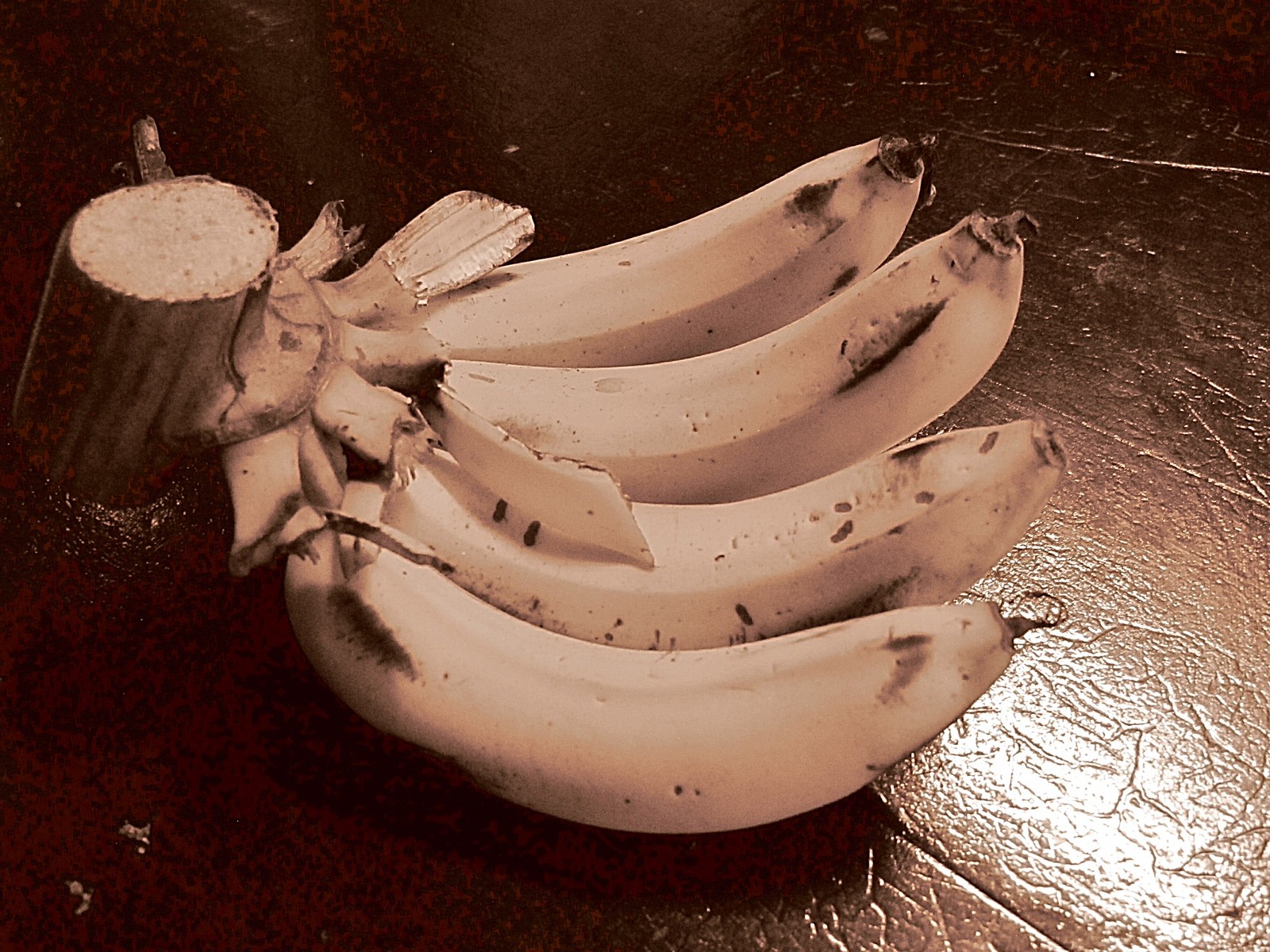This photograph captures a natural setting on a wooden surface, which could be either a floor or a table. Dominating the image is a seemingly freshly-harvested bunch of bananas, still attached to a sizable tree branch, approximately two to three inches in diameter. Unlike the typical store-bought bunches, this one has a rustic, straight-from-the-tree appearance. 

The bunch appears to have been recently cut, showcasing some partial peels on the top layer, suggesting that three to four bananas have already been removed. The remaining bananas, possibly numbering eight to ten, are mostly off-white with noticeable brown and black specks, indicating varying stages of ripeness. The ends of these bananas show small, dried-up growths, further emphasizing their natural, unprocessed state. The vivid contrast between the wooden surface and the bananas accentuates the organic texture, making the scene appear both rustic and fresh.